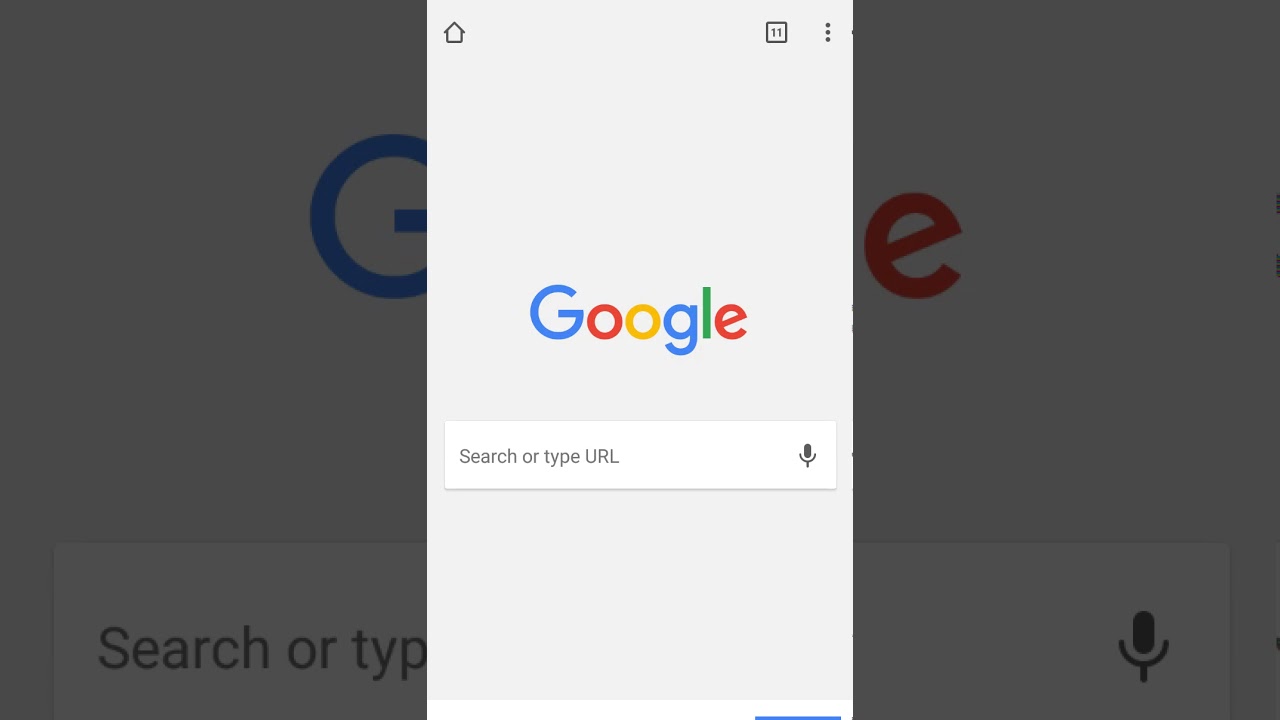The image features a computer screen in the background with the Google home page partially visible. The screen prominently displays the uppercase "G" and the last "E" of the Google logo, along with the search bar which reads "Search or type" and a microphone icon on the far right. Dominating the center of the background is a gray rectangular pop-up window. At the top of this rectangle is a home icon, followed by a small square with the number "11" in it and three vertical dots. In the middle of the gray rectangle, the colorful Google logo stands out, with a blue capital "G," a red first "O," a yellow second "O," a blue lowercase "g," a green "l," and a red "e." Below the logo is a white search bar that reads "Search or type URL," with another microphone icon on its right side. The bottom of this pop-up area is white, and a small blue line is visible along the edge on the right side.